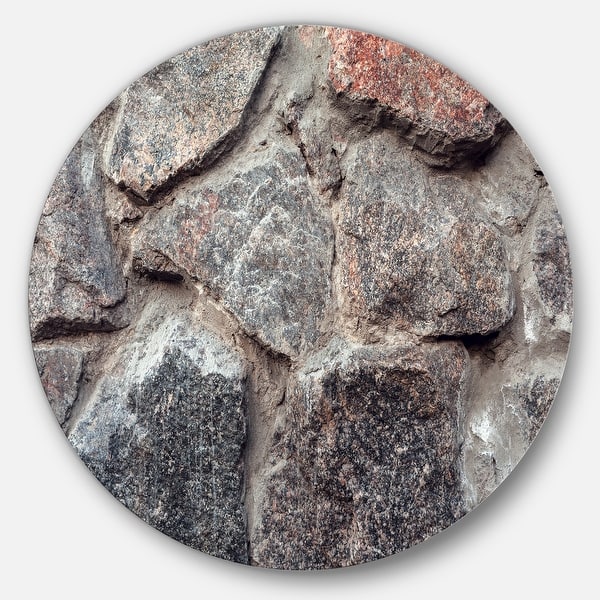The image depicts a meticulously crafted circular stone display piece, set against a light, almost white or beige background. The perfectly round structure is made from various types of stones seamlessly fused together, with an intriguing array of colors and textures. Prominently, there is a red stone at the top right, bordered just below by a lighter gray stone with subtle shading. A series of darker stones follow, interspersed with lighter stones that exhibit nearly golden hues towards the upper part. The stones exhibit a natural assortment of colors, including shades of gray, black, brown, and white, creating a mosaic-like pattern that showcases both uniform and irregular shapes. The overall composition suggests an artistic and possibly purchasable display piece, emphasizing the seamless merger of natural elements.